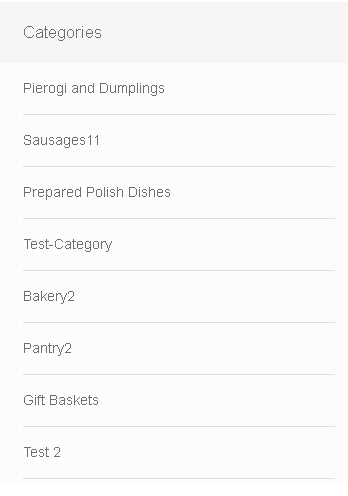The image features a selection box containing a list of 10 categories, with one main category and 9 subcategories positioned underneath. Each category is presented within white boxes separated by horizontal lines, extending from left to right.

On the left-hand side, there is a gray horizontal box featuring categories in a thinner, typewritten text. The following is a detailed description of each item in the list:

1. **Pierogi and Dumplings** - Listed with capital 'P' and 'D'. The first item in this subcategory.
2. **Sausages11** - Presented with a capital 'S' in 'Sausages' and immediately followed by the number '11' with no spacing.
3. **Prepared Polish Dishes** - Each word starts with a capital letter.
4. **Test-Category** - Written without spaces, with 'Test' having a capital 'T' and 'Category' with a capital 'C'.
5. **Bakery2** - Capital 'B' for 'Bakery' followed by the number '2' without any spaces.
6. **Pantry2** - Similar style to the Bakery2 entry, starting with a capital 'P'.
7. **Gift Baskets** - Each word with a capital 'G' and 'B'.
8. **Test 2** - A space between 'Test' and '2', with 'Test' starting with a capital 'T'.

Overall, the image is organized with a visually distinct layout, utilizing clear text formatting to separate and categorize each item.